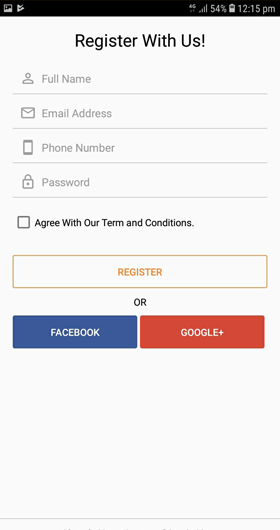The image depicts the registration section of a website as seen on a mobile phone. At the top of the screen, the time is displayed as 12:15 PM, and the battery level shows 54% charge. The header, titled "Register with Us," is positioned below a small black, skinny rectangular strip that contrasts with the white background of the registration form. 

This registration form is organized with several input fields labeled "Name," "Email Address," "Phone Number," and "Password." Below these fields, there is a checkbox option to "Agree with our Terms and Conditions."

The registration button at the bottom stands out with its orange text on a white background, framed by a thin orange border. Alternatively, users can choose to register through social media options. Between the standard registration box and the social media options, the word "or" is displayed, providing a separator.

Two social media options are available: a Facebook registration button, featuring white text on a blue background, and a Google Plus button, displaying white text on a red background. Each button is bordered by a faint gray line at the very bottom, reinforcing the section's clean and organized layout.